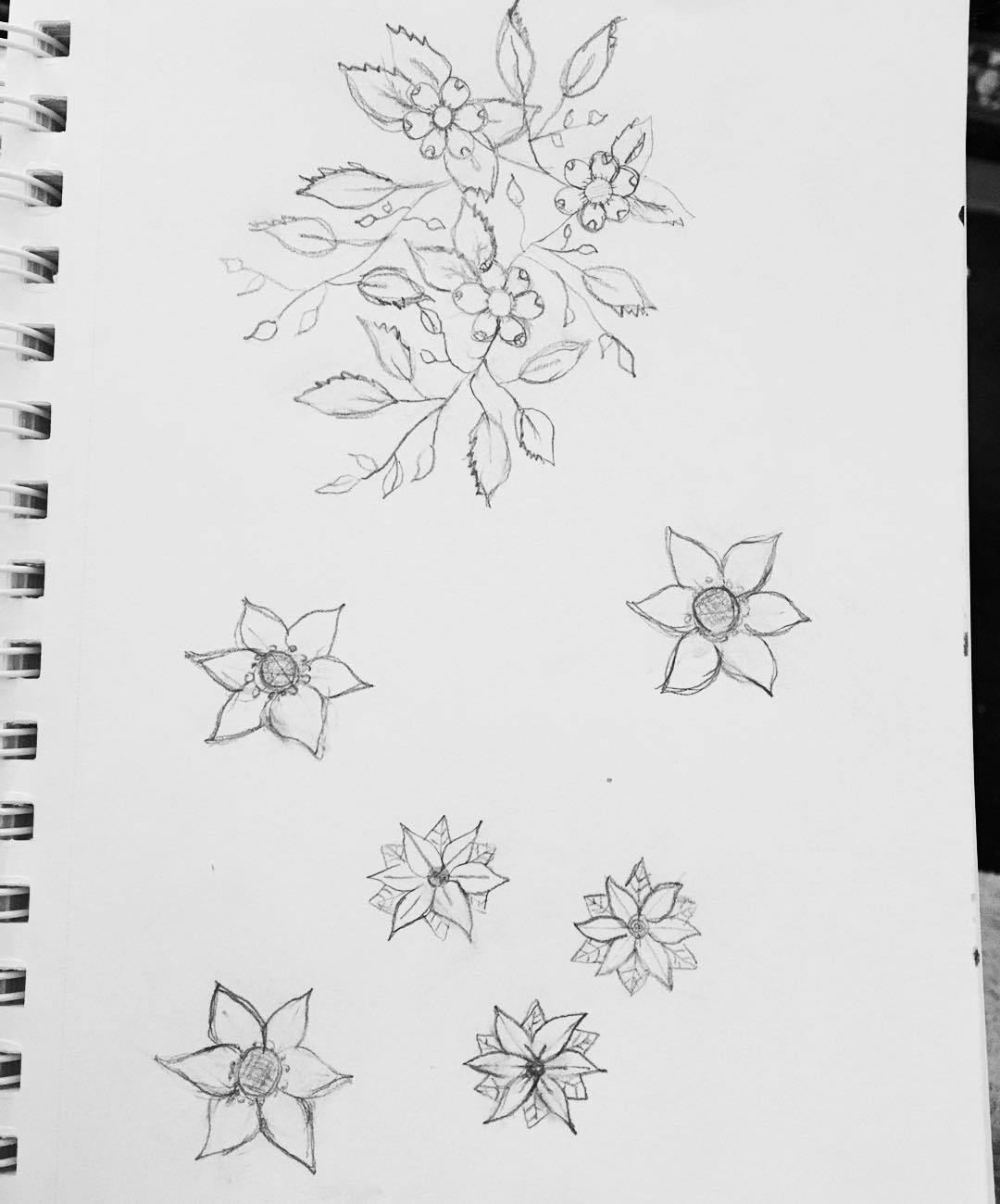This is a detailed black-and-white pencil drawing on a white sheet of drawing paper, bound in a notebook with visible rings on the left side. The drawing features two main sections of floral sketches. The bottom half displays six simple flowers: three smaller ones arranged in a triangular pattern with six distinct petals, each framed by six darker, more detailed leaves. Surrounding these, three larger flowers also with six petals add variation, though the petals remain simple and unornamented.

In contrast, the top half of the drawing showcases a more intricate design. It features a cluster of three flowers with rounded petals, accompanied by branches that weave into a web-like structure. These branches bear detailed leaves with visible veining, smaller buds poised to bloom, and heavily shaded flower centers, demonstrating more complexity compared to the bottom section. The entire sheet includes small pencil marks scattered across, enhancing the sketch-like, artistic feel of the drawing.